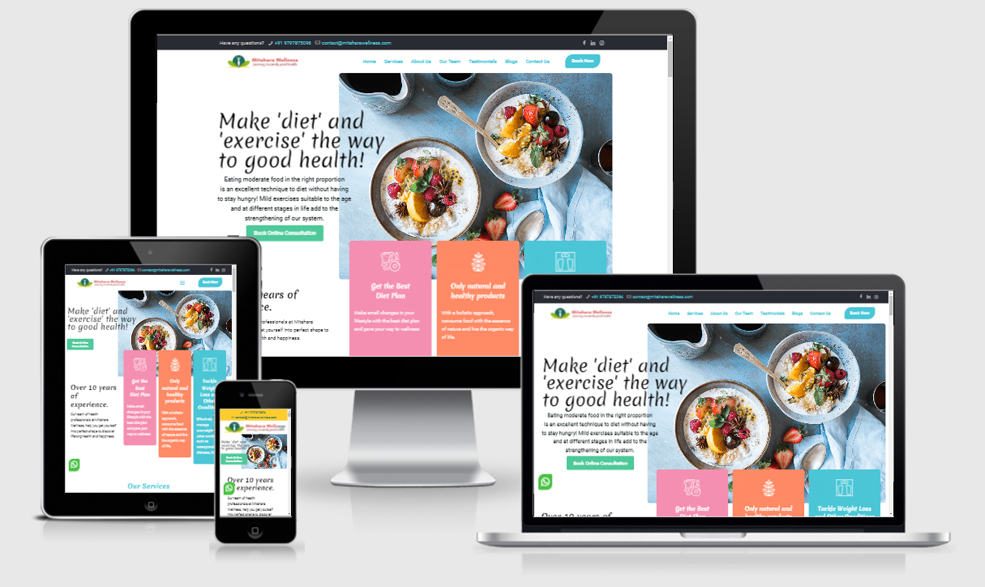This image showcases a website prototype being tested across multiple devices. Four digital devices are displayed, emulating a common setup for responsive web design testing. Prominently featured is a digitally drawn MacBook, paired alongside a stand-alone monitor. To the right of this setup is a sleek MacBook Air, known for its thin profile. On the left side of the image, an iPad with a characteristic black bezel and a small square home button is visible, indicative of typical iOS design. Directly below the stand-alone monitor, an iPhone featuring the same black bezel and home button as the iPad completes the array of devices.

Each device displays the same website, allowing for a comparative view of its responsive design. The desktop and MacBook iterations exhibit a consistent layout, with a clean white space evident around content sections. The tablet version appears more compact, with elements condensed to fit the smaller screen, leading to a more crowded visual. The mobile variant presents the most significant adaptation, with the main image scaled down and ancillary content boxes omitted, likely accessible through scrolling.

The website content focuses on promoting health through diet and exercise, as indicated by the prominent headline, "Make diet and exercise the way to good health." The site features vivid images of healthy food, supporting the wellness theme. Navigation links span the top of each device’s screen, and a conspicuous registration button sits in the top-right corner, inviting user interaction.

Overall, the image captures a detailed look at how a health-focused website adapts across various digital platforms, emphasizing the importance of responsive design.